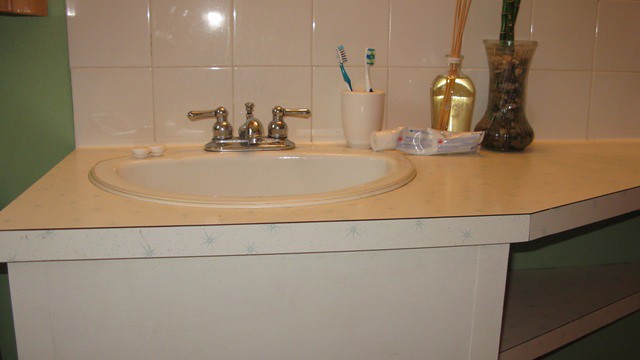This photograph captures an authentic 1970s-style bathroom sink area in meticulous detail. On the far left of the image, a bright green wall adds a splash of vibrant color to the setting. The background features shiny white ceramic tiles arranged in a square pattern, giving the space a classic touch. The countertop, made of old white Formica, is adorned with a subtle light blue splatter pattern, exuding a vintage charm. 

The sink itself is rimmed and inset, complemented by a faucet with two brass-plated handles that gleam under the light. To the right of the sink, a white ceramic toothbrush holder stands, containing two toothbrushes standing upright. Adding a touch of modernity, a scented oil container with reeds protruding from it sits nearby. Next to this, a small vase, possibly containing a cactus, lends a hint of greenery to the scene.

A well-used tube of toothpaste lies close to the sink, noticeably squeezed to the brink of emptiness. The countertop angles off to the right and towards the back, where it joins a cabinet featuring two drawers directly beneath it. This detailed arrangement provides a nostalgic glimpse into a distinctly styled era.